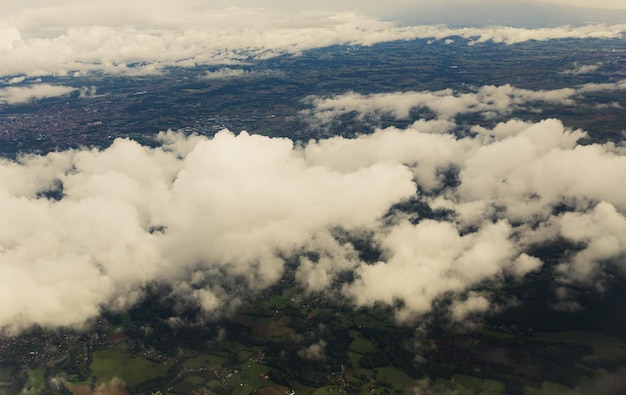An aerial photograph, likely taken from an airplane, captures a breathtaking view above the cloud layer, revealing a sprawling rural landscape below. Puffy white clouds drift across the image, creating gaps through which the verdant country scenery, characterized by a patchwork of green fields, dense tree clusters, and small towns, is visible. The foreground features these clouds prominently, giving way to a clearer view in the middle of the image, where the landscape stretches far into the distance. At the top of the photo, a long strand of clouds stretches horizontally across, adding depth and perspective to the scene. The photograph, taken during the day, has a nostalgic feel, perhaps due to a filter that imparts a subtle yellow tint, contrasting with a bluish hue in the top right corner, lending an old-fashioned charm to an otherwise clear and crisp image.